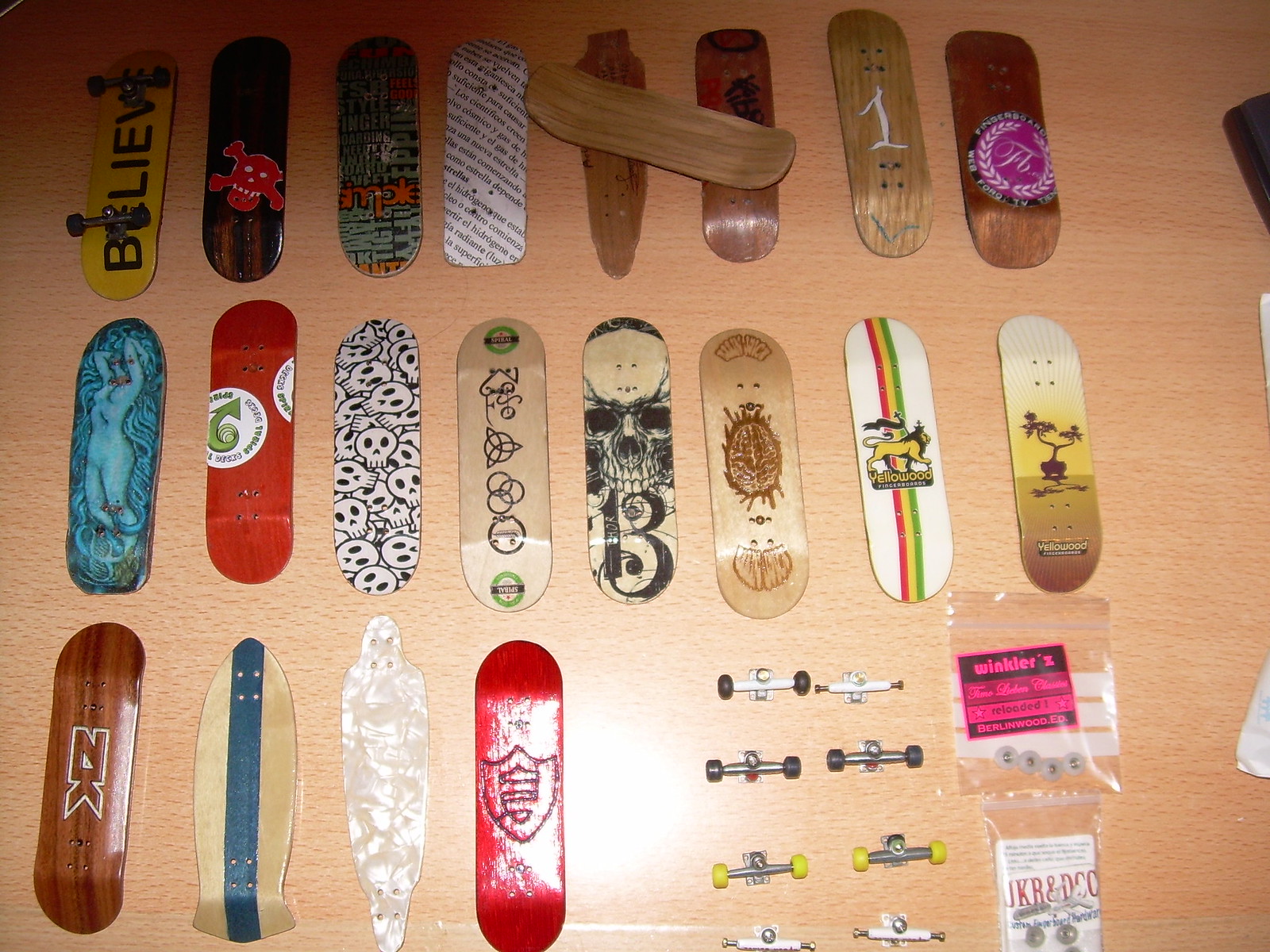The image displays a meticulously arranged collection of approximately 20 miniature skateboards, or fingerboards, mounted on a salmon-colored wooden wall. These fingerboards feature a variety of intricate and vivid designs, including wood tones, red, white, turquoise, purple, green, and yellow. Prominent among the designs are two boards with skull motifs and one with the word "Believe" inscribed on it, alongside another board labeled "Yellowwoods." The fingerboards are arranged in two rows of eight and one row of four. Several boards appear to be made of wood, while others are plastic or pearlescent materials. Some boards have trucks and wheels attached, either in black or neon yellow, while additional skateboard trucks and wheels are mounted separately on the wall. The image also includes some papers and bags of wheels, emphasizing the theme of customizable skateboard parts.